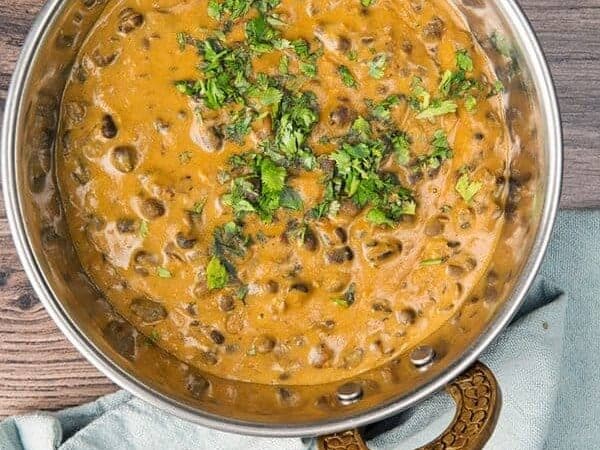The image is a detailed, overhead, close-up view of a silver pot containing a thick, creamy orange-brown stew or porridge. The stew appears to have beans scattered throughout, adding a slightly darker brown contrast to the base. Sprinkled on top are green herbs, which may be chives, basil, or rosemary. The pot features copper or leather-like handles, bolted onto the sides. It rests on a wood grain table, with part of a white towel visible beneath it on the right side. The photograph's composition, showcasing these various textures and ingredients, suggests it could be used for a cooking site accompanying a recipe.